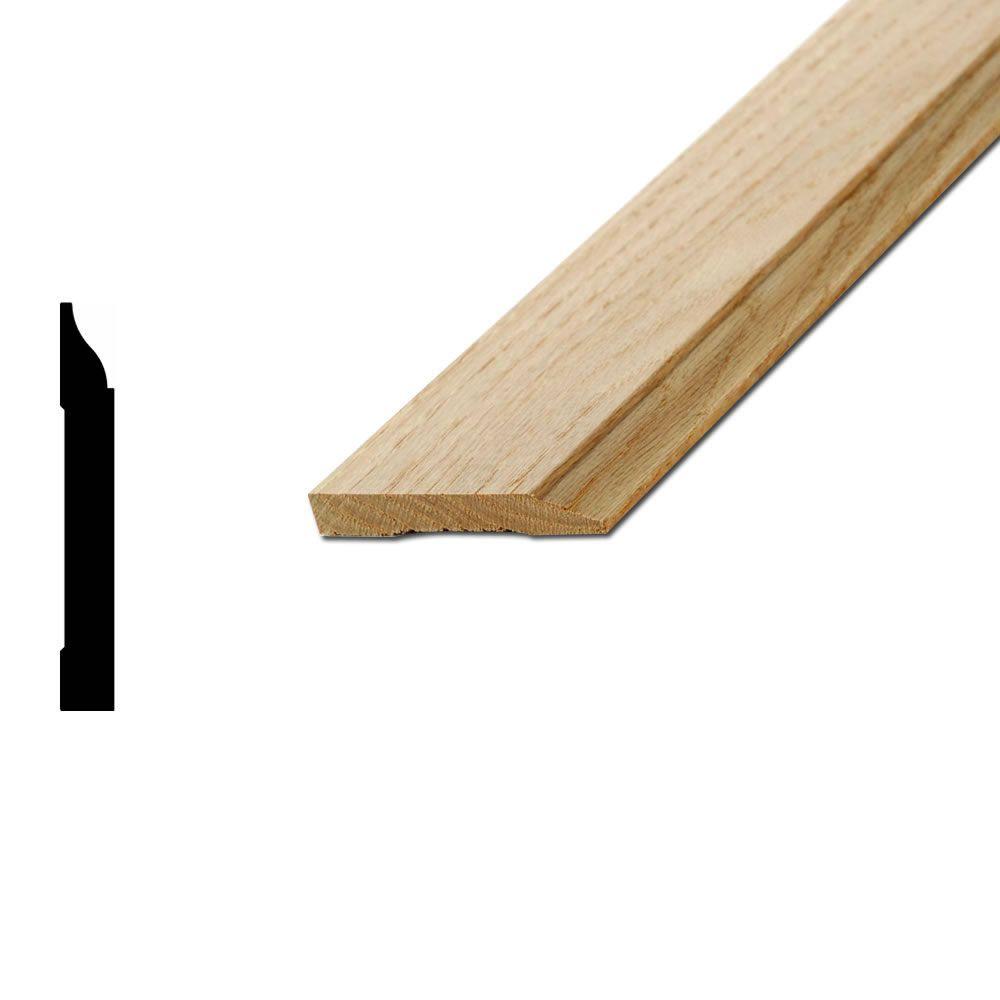The image features a piece of lightweight, light brown plywood with distinctive medium to dark brown wood grains traveling vertically. This piece of wood diagonally descends from the upper right corner towards just past the middle of a solid white background, ultimately exposing its flat, beveled end as it approaches the lower left quadrant. The plywood resembles a shelf or possibly molding due to its beveled edge. Notably, on the lower left side of the image, there is an ambiguous black shape reminiscent of a paintbrush or a bar, with a rectangular base and a curved, pointed tip. The shape is solid black and lacks any discernible label or text.